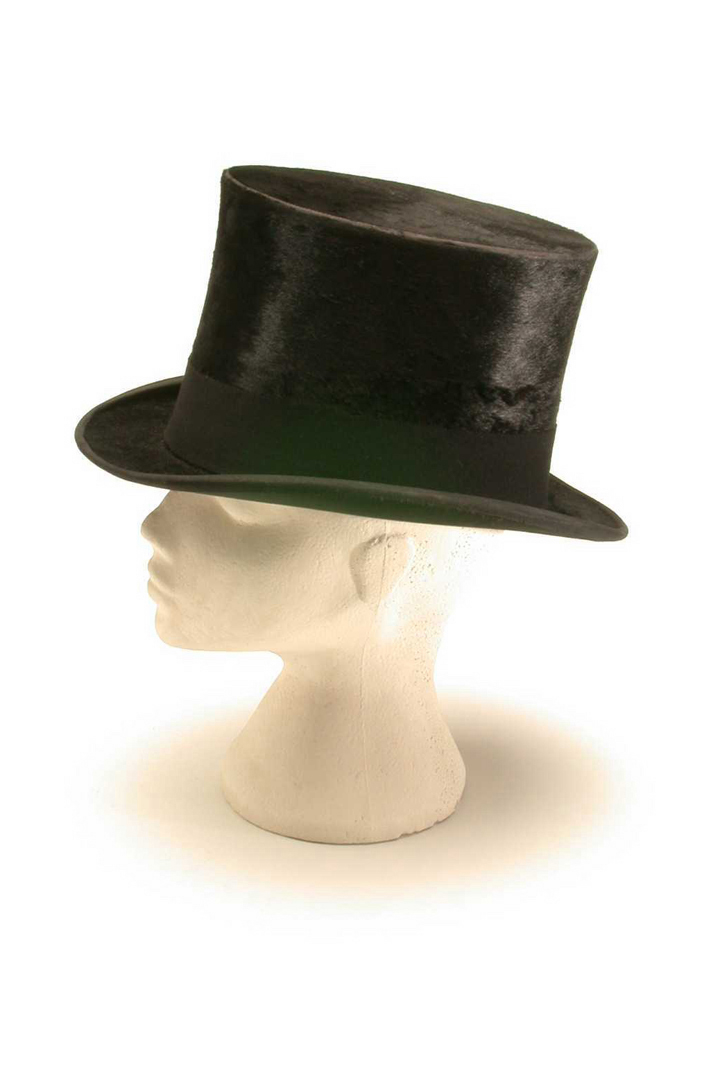This image showcases a white mannequin head with a neck, prominently featuring a visible seam running from the ear down to the neck on the side. Positioned with its face turned to the left, the mannequin displays shadows under the eye, over the top of the nose, and towards the back right of the neck, adding depth and contrast. The mannequin is adorned with a black top hat made of a velour-like material. The hat's rim subtly curves upward on what appears to be the front left side. Reflecting off the rim of the hat, an off-white light can be seen beneath the mannequin, adding a touch of brightness to the overall composition.